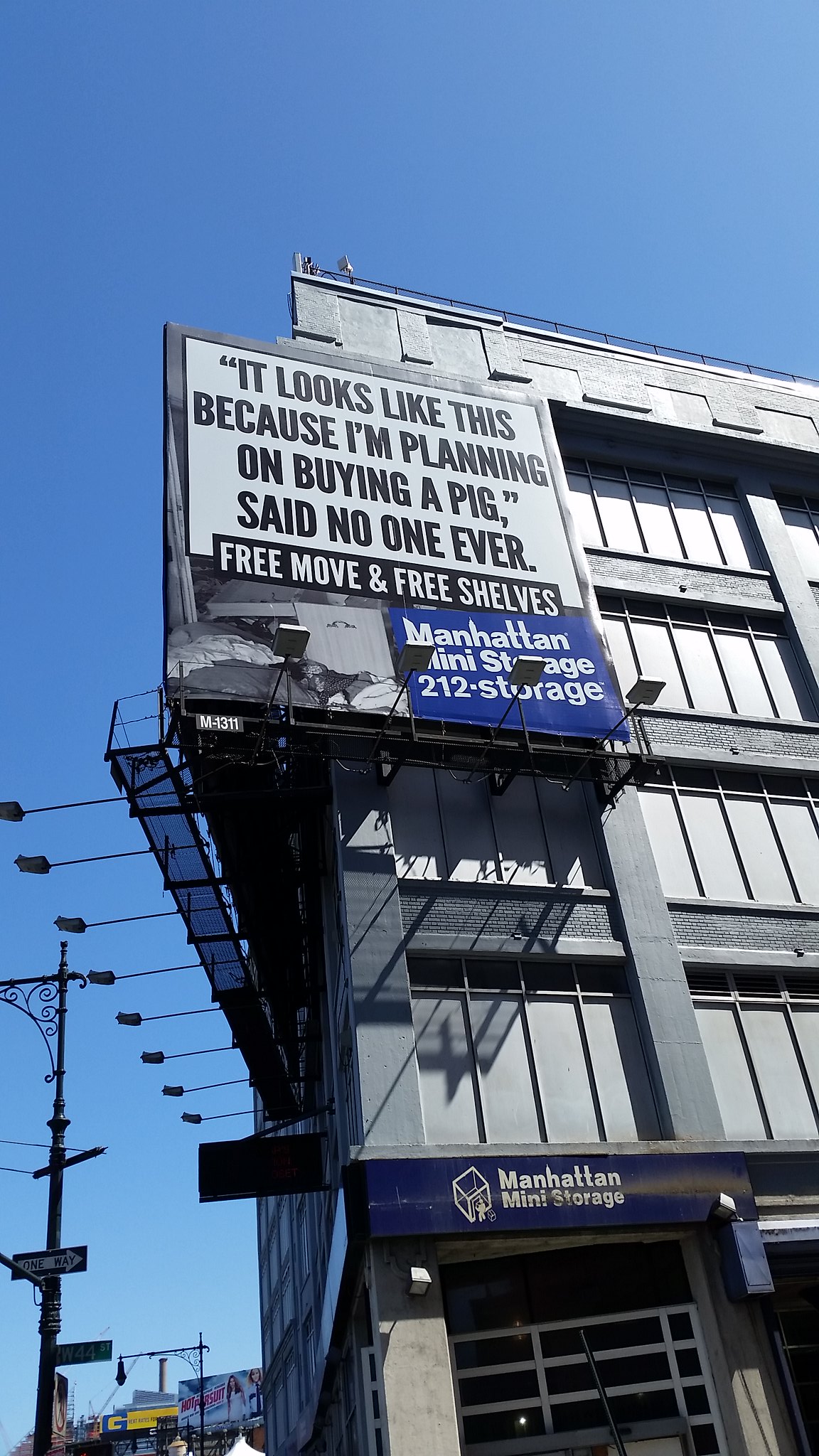In this photograph taken on a clear, sunny day with a medium blue sky, the viewer looks up at an older gray building, which stands at least five stories tall and prominently features "Manhattan Mini Storage" signage at the ground level. The building is characterized by its large, gray-framed windows and gray columns, with an intricate scaffolding walkway visible at the top left. A notable advertisement atop the building, with a gray frame, white background, and black letters, humorously declares, "It looks like this because I'm planning on buying a pig, said no one ever." Beneath this, the ad offers "Free move and free shelves" and lists the storage facility's contact as "Manhattan Mini Storage, 212-STORAGE," presented in a blue box with white lettering. To the left of the building, a black-and-white One Way street sign points to the right, situated on a pole with affixed lights, but another green street name sign remains illegible. Additionally, there's a small image of a messy room depicted on one of the billboards below the main advertisement.